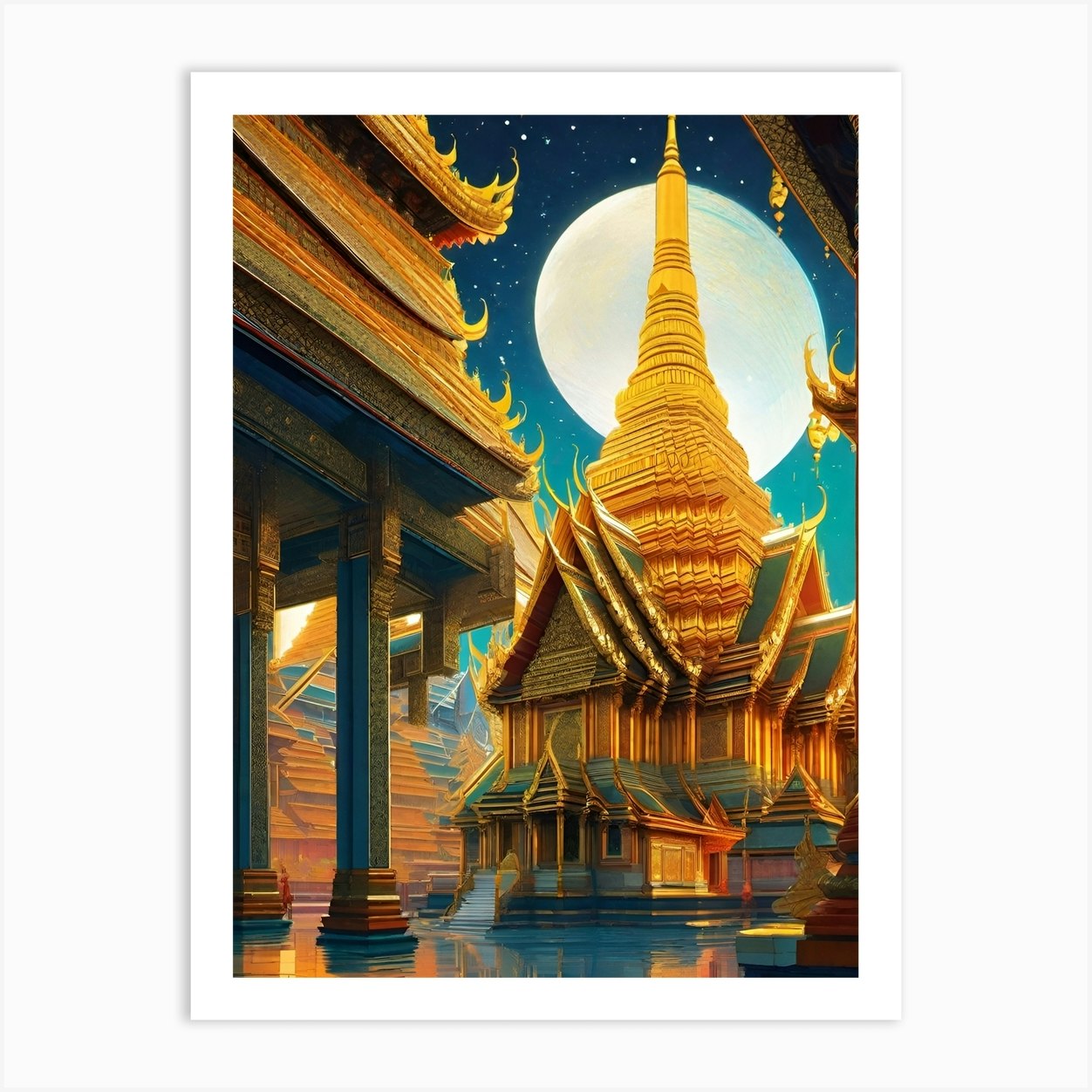This image depicts a detailed, dreamlike painting of a night scene showcasing a golden Buddhist temple complex, likely inspired by Thai architecture. The central feature is an ornate temple with a tiered roof and a tall, multi-layered spire reaching towards the sky. The roof lines of all the buildings in the painting curve upwards in elaborate tiers, exhibiting typical Southeast Asian design elements. The night sky serves as a serene backdrop, awash in shades of deep blue and turquoise, and featuring a large, somewhat oblong full moon emitting a soft yellow-orange glow. The buildings themselves are predominantly golden yellow, adorned with splashes of green and orange. The entire scene is framed by a white border, adding a touch of modernity to the classical beauty of the temple. The perspectives in the painting are slightly off, especially around the front entrance, hinting that it might be AI-generated. Overall, the painting exudes a sense of tranquility and perfection, akin to a travel poster or postcard showcasing an idyllic, nocturnal view of a Thai pagoda.